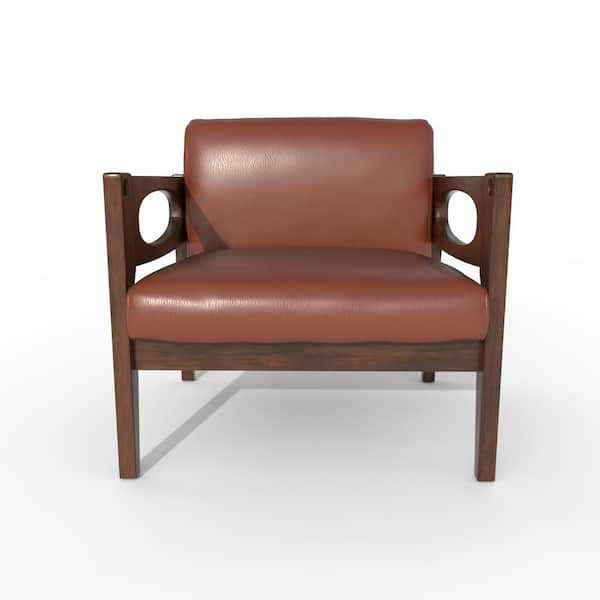This image depicts a brown armchair with distinct features and set against a minimalist background. The chair is oriented directly towards the viewer, with a stark contrast between its rich hues and the plain backdrop. The background transitions smoothly from light gray at the bottom to white at the top, suggesting a simple surface upon which the chair is placed.

The armchair itself has a robust wooden frame characterized by dark brown wood on its four sturdy legs and armrests. Notably, the armrests are adorned with circular cutouts at the sides and connected by a horizontal strip of wood across the front. The seat and back cushions are wide and share the same medium brown color, a leather or vinyl material that complements the darker wooden frame.

The setting is devoid of any additional objects, text, or figures, emphasizing the singularity of the chair. The photograph is taken from a straightforward perspective, capturing the chair's full structure and details, including subtle shading and shadows beneath it. The armchair stands out as the focal point in an otherwise empty and pristine environment, highlighting its design and craftsmanship.